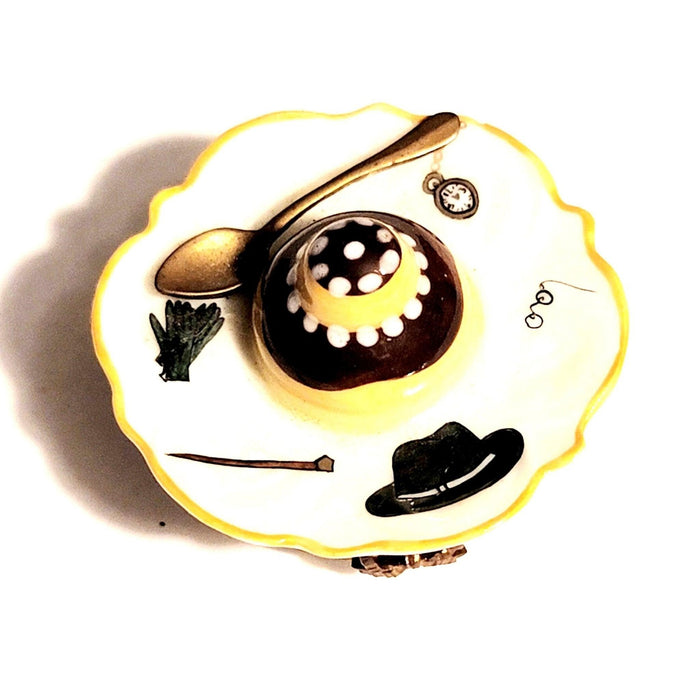This is a top-down photograph of an intricately designed serving plate with a distinctive yellow border. The center of the plate features a series of concentric circles: starting with a white ring, followed by a yellow ring, a black ring with white polka dots, another yellow ring, and culminating in a black center also adorned with white polka dots. Placed on the upper left portion of the plate is a silver spoon, oriented such that the handle points upwards and the bowl downwards. The white section of the plate is decorated with detailed illustrations, including a pocket watch, a pair of gloves, a walking cane, a black fedora hat with a white ribbon around the base, and a pair of fancy eyeglasses with a string attached. The design elements suggest a vintage or elegant theme. At the bottom of the image, a brown object partially peeks out from behind the plate, though its identity is unclear. The plate casts a dark gray shadow to its left, adding depth to the image. Additionally, there is a small black dot located directly below and to the left of the plate on the table. The overall presentation is clean and unique, with the possibility that the spoon and other elements might be part of an edible arrangement, such as a cake.